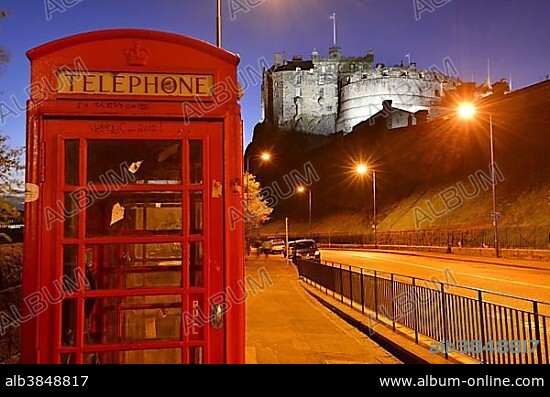The full-color photograph, taken shortly after sunset, features a square layout with no definitive border except for a black bar at the bottom displaying the text "ALB3848817" on the left and "www.album-online.com" on the right. The background bears a digitally added watermark that repetitively says "album." Off to the left side of the image stands a classic British red telephone booth with glass doors and a rectangular white sign labeled "telephone" at the top. The booth is situated on a sidewalk next to a black metal railing.

The scene is set against a darkening sky, a rich blend of dark blue and dark purple hues, indicating the nearing of nighttime. A road runs parallel to the sidewalk, flanked by street lamps casting an amber glow on the pavement. A few cars are parked along the side of the road. In the distance, a steep, green hill ascends sharply into the frame, atop which stands a grand, gray stone castle, illuminated by spotlights that highlight its towering walls and rounder sections. Flags and flagpoles are visible, accentuating the fort-like appearance of the structure.

Overall, the photograph captures an intriguing blend of natural and artificial lights, with the picturesque telephone booth in the foreground juxtaposed against the majestic, spotlit castle on the hill in the background.